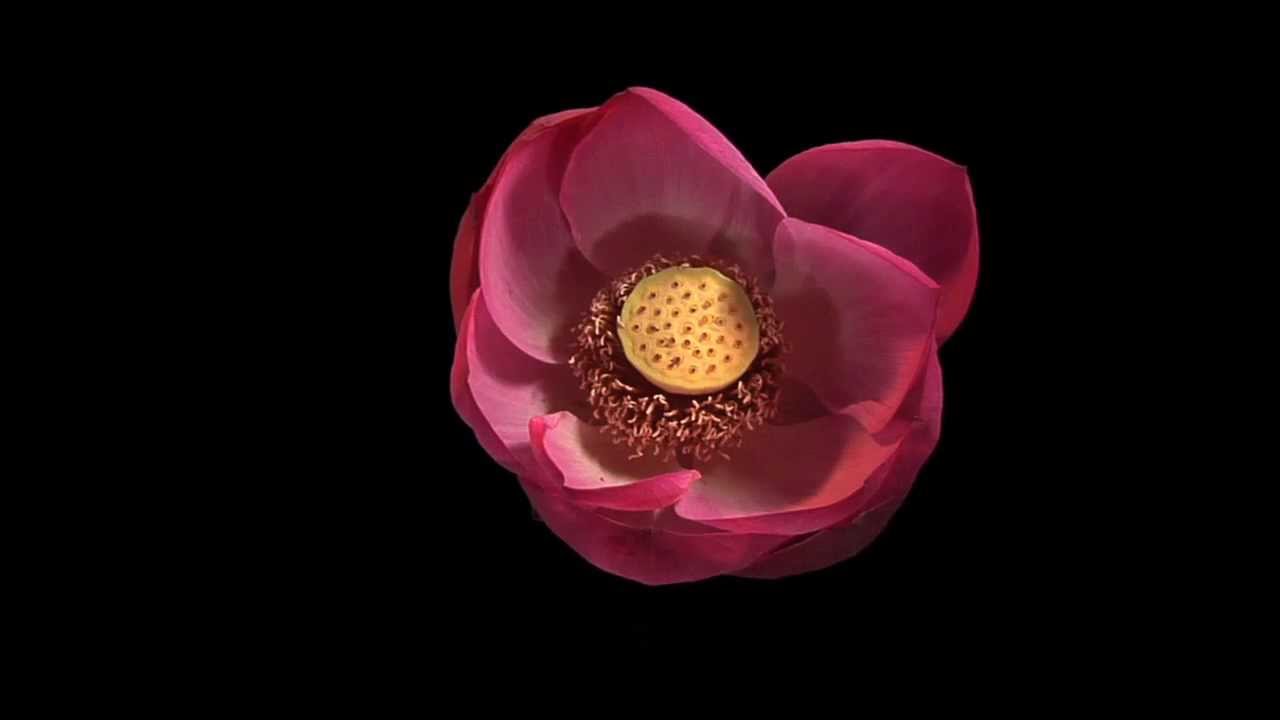This is a detailed close-up image of a reddish-violet flower set against a plain black background. The flower, viewed from the top, showcases its intricate petals and center in stunning clarity. The petals are fine, thin, and soft-looking, with a color gradient that transitions from a creamy white at the base to a deeper reddish-pink at the edges. These petals, wider than teardrops, exhibit a slightly spade-like shape, with some curling at the edges and one petal conspicuously bending in towards the center.

The heart of the flower features a central yellow-green circle, possibly representing the main pollen area, adorned with numerous tiny red dots. Surrounding this center are slender, rice-like structures that appear almost furry, comprising white and red-tinted segments. The petals are arranged in a layered formation, creating a staggered, cup-like arrangement, reminiscent of a rose or tulip. Despite the absence of the stem and leaves, the detailed depiction of the flower's head against the stark black background highlights its striking beauty and vivid colors.